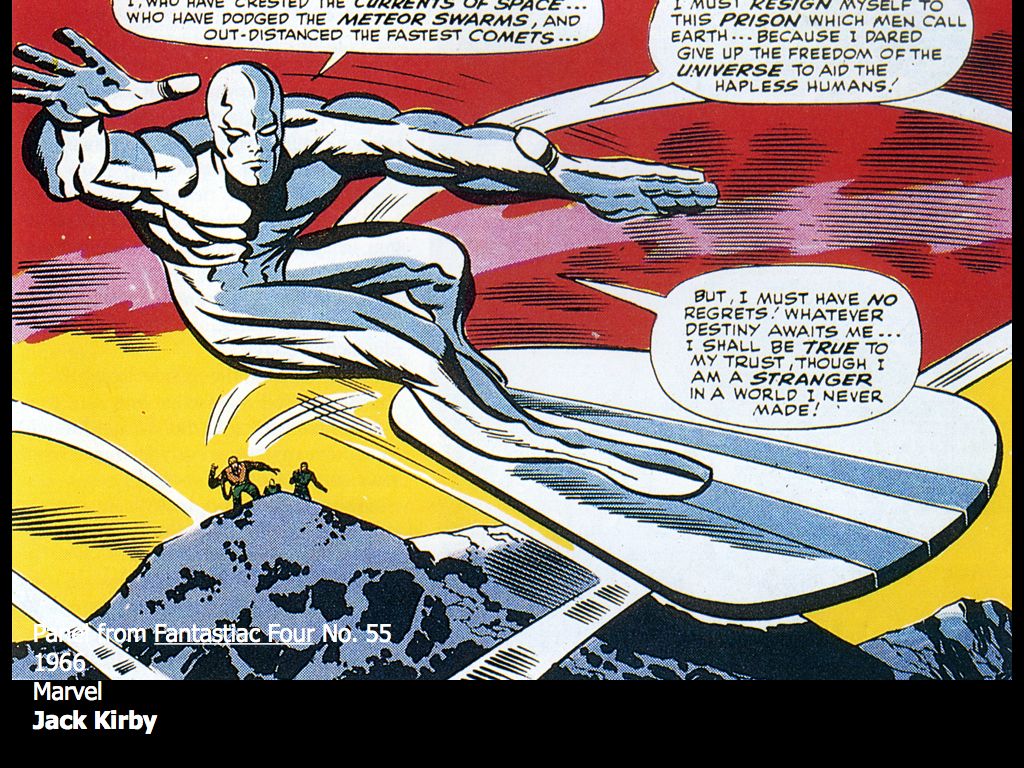In this comic book panel from Marvel's Fantastic Four number 55 (1966), created by Jack Kirby, the Silver Surfer soars through a red and yellow sky on his iconic surfboard. The top of the panel cuts off two dialogue bubbles, which continue to describe his inner turmoil. Below him, a mountain range stretches across the bottom of the image, with several men visible on a mountaintop. The full dialogue in the panel reads, “But I must have no regrets. Whatever destiny awaits me, I shall be true to my truest trust, though I am a stranger in a world I never made.” The artwork is bordered by thin black lines on the left and right, while the bottom left corner features the letters “PA,” and text that reads “Fantastic Four, number 55, 1966, Marvel, Jack Kirby.” The vivid colors and dramatic composition capture the essence of the Silver Surfer's cosmic journey and existential conflict.